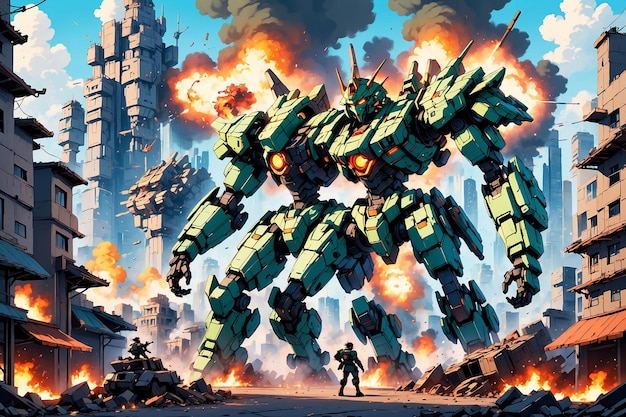The image appears to be a dramatic scene from a modern comic book or animated series, featuring a chaotic futuristic urban landscape under attack. Dominating the scene are two enormous, light green, transformer-style robots with glowing orange or yellow light emanating from their chests, likely a combat feature. Although they have a combined total of three and a half legs and are connected at the shoulder, suggesting they might be merged or improperly rendered, one of them has a head adorned with spikes and glowing eyes. Amidst the explosions and fires consuming several buildings, a soldier stands defiantly on the rubble-strewn ground, engaged in battle. Nearby, a small yet sturdy vehicle with a human operator inside also aims its weapon at the colossal adversaries. The backgrounds illustrate the extensive destruction, with multiple structures crumbling and engulfed in flames, creating an intense atmosphere of warfare and ruin.